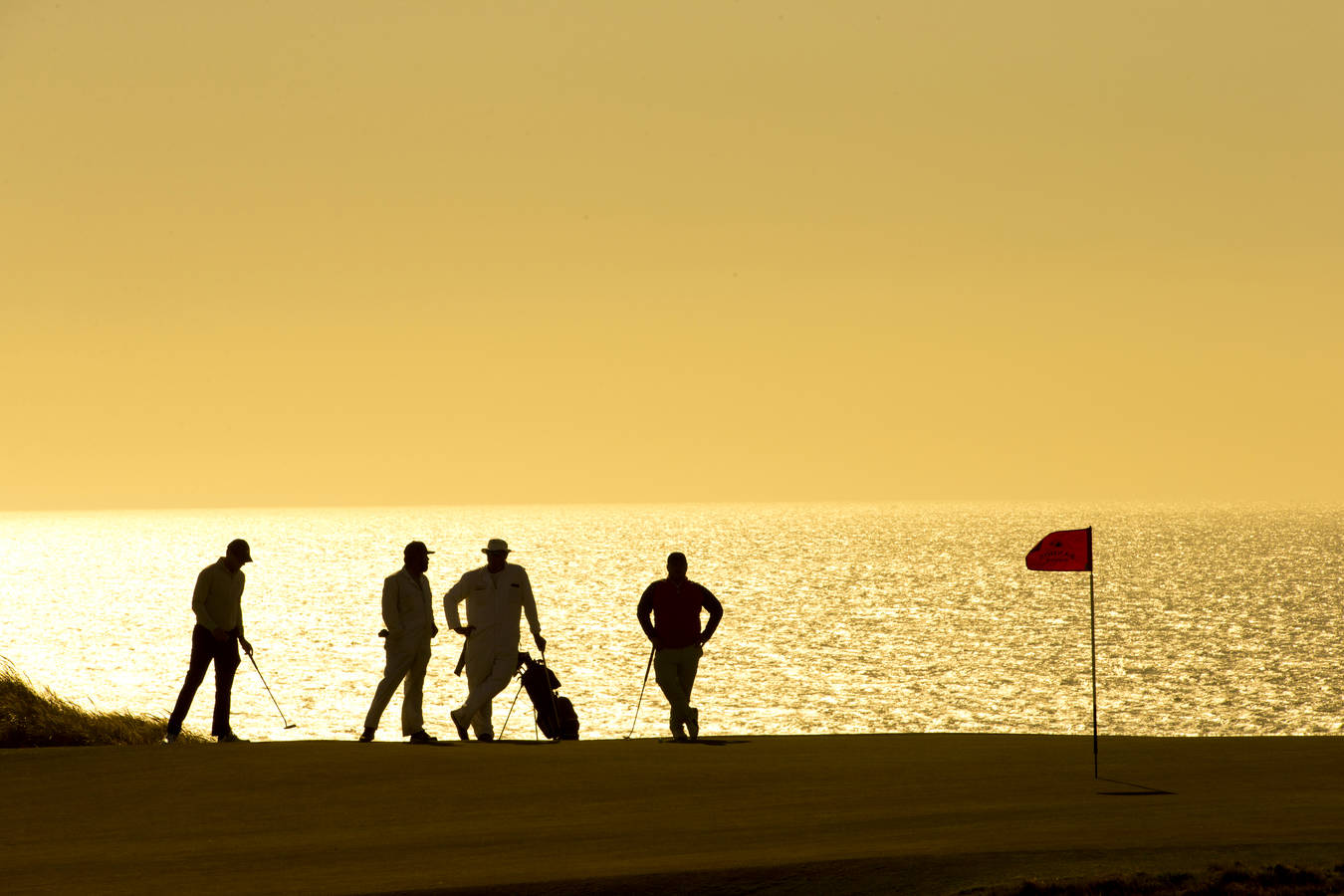In this striking color photograph captured at sunset, a group of four silhouetted golfers pauses to admire a breathtaking scene. They stand on a gently elevated hill of a golf course, with the putting green outlined against a vast, calm body of water, possibly an ocean. The sky and water are both tinted a mesmerizing yellow-orange hue, casting a warm golden glow over the scene. 

One golfer, distinguishable by his stance, gazes contemplatively out over the water, resting on his golf club. Another golfer approaches, seemingly eager to share in the view. Nearby, two other men, also leaning on their clubs, are engaged in quiet conversation. Among the group, three wear hats—two baseball caps and one of a different style—while the fourth man remains hatless. 

A vivid red flag flutters gently in the breeze, secured in the cup on the putting green. Beside the group, a golf bag rests on a small two-stand contraption. The tranquil, golden-hued scene encapsulates a serene moment of camaraderie and reflection amidst a game of golf by the water.